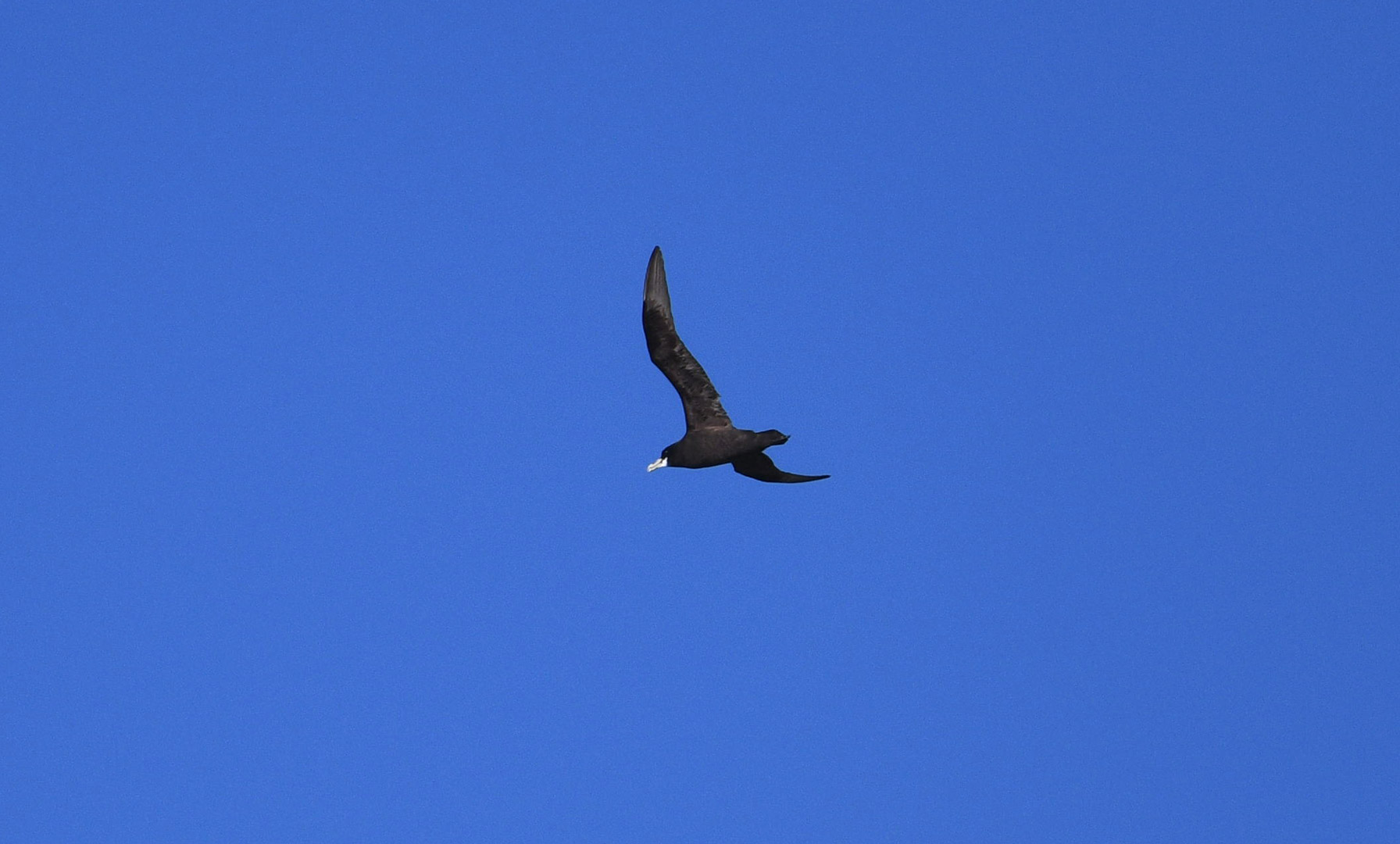In this image, a lone bird soars gracefully in a clear, bright blue sky devoid of any clouds or other elements. The bird, which is possibly a seagull or another species of similar size, appears predominantly black with striking grayish or silver streaks near the tips of its widespread wings. A white beak or "beard" adds contrast to its otherwise dark plumage. The bird’s tail feathers are straight out as it glides effortlessly, suggesting it is more likely gliding than actively flapping its wings. Its exact size and species remain unclear due to the absence of any reference points in the sky, but the vivid clarity of the daylight and the serene expanse of the azure sky encapsulate the bird’s tranquil flight.